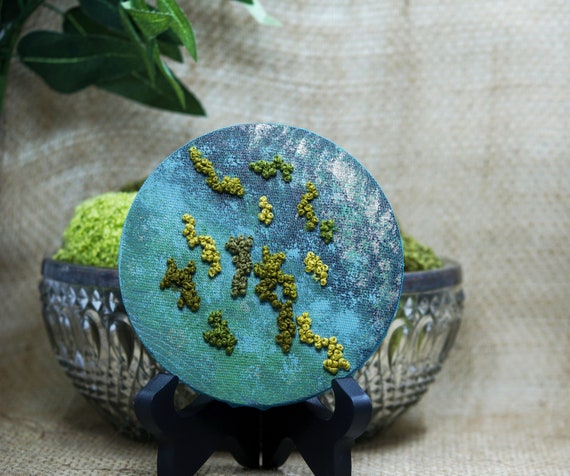The image features a detailed artistic display set against a cream and light brown canvas backdrop. In the upper left corner, green leaves hang down, adding a touch of nature to the scene, while the upper right, lower right, and bottom exhibit the plain light brown canvas. Central to the image is a meticulously crafted embroidery piece, held by a dark blue wooden holder with three legs and two arms. The embroidery hoop contains a circular canvas painted in various shades of blue, evoking the appearance of a globe with white and green accents. Adorning the blue canvas are clusters of green, yellow, and dark green French knots, potentially representing islands or geographical features. Below this artistic globe, a blue and silver metal bowl sits, possibly containing green objects, hinting at materials used in the creation of the piece. The overall setting presents a harmonious blend of colors and textures, showcasing an intricate embroidery work, which could well be aimed at displaying craftsmanship for potential sale, reminiscent of items seen on platforms like Etsy.